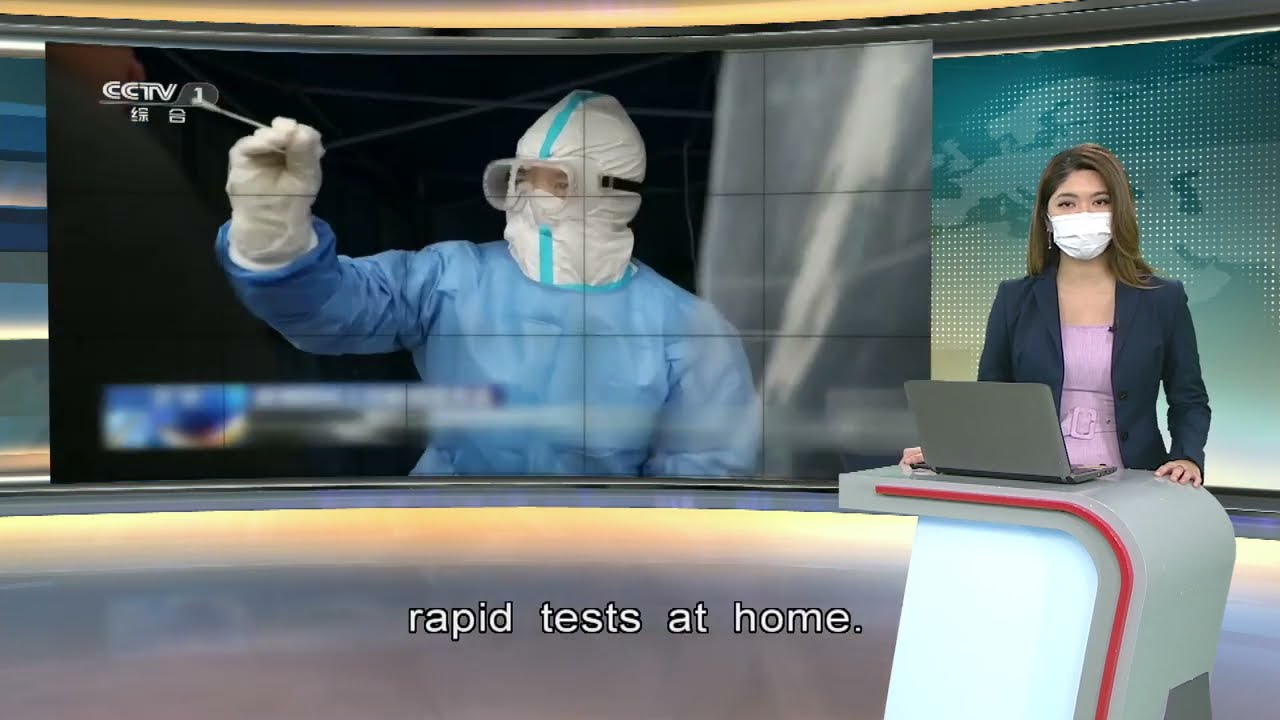The image depicts a detailed screenshot from a news broadcast. In the foreground stands a young Asian woman, likely in her 20s or early 30s, serving as the news anchor. She has long brown hair and is dressed in a blue blazer over a pink top, detailed with a belt. A white mask covers her face. In front of her is an open gray laptop, placed on a custom-made podium characterized by a gray surface with a round edge and a red line running through its middle.

The backdrop features a green, digitally-rendered world map with a headline that reads "rapid tests at home." To the anchor’s right, the screen shows an image from CCTV of a healthcare worker or possibly a scientist, entirely clad in a blue hazmat suit, complete with gloves, goggles, and a protective face mask. The individual is holding out a nose swab, likely demonstrating a COVID-19 rapid test. This comprehensive setup suggests that the newscast is covering health-related topics, possibly during the COVID-19 pandemic.